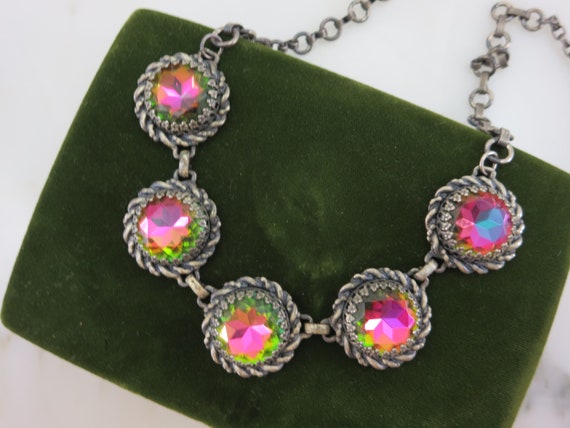The image showcases a necklace made of a slightly tarnished silver chain, prominently displaying five large, spherical gems. Each of these gems exhibits a vibrant interplay of colors, reflecting mainly pink, green, and orange hues. The rightmost gem specifically radiates a combination of pink and blue light. This striking necklace is meticulously arranged on a luxurious green velvet cushion, positioned at an angle against a starkly white background. The velvet stand accentuates the bright, multi-colored gems, which may or may not be genuine precious stones. Despite some ambiguity about its exact nature, the overall presentation suggests that the necklace is designed to catch the eye of potential buyers, possibly in a store setting where it is being showcased for sale.